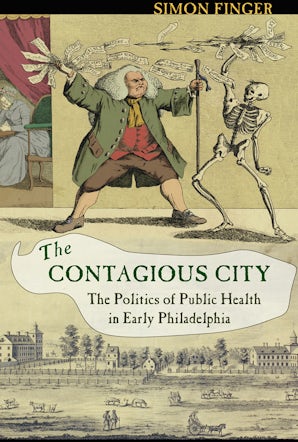This is an image of a colorful book cover isolated on a white background, featuring a vertical rectangular design. At the top of the cover, there is a black horizontal bar, with the author's name, "Simon Finger," in yellow text on the far right upper section. Below this bar, the central illustration depicts a man in 18th-century attire, reminiscent of Benjamin Franklin, with a white wig, a long frock coat, a red waistcoat, brown breeches, brown stockings, and buckle shoes. He faces and seemingly battles a skeleton, both clutching slender strips of paper between them. Additional details include a black and white drawing beneath the main image, showcasing an early Philadelphia cityscape with the Delaware River, featuring boats, people in period clothing, various buildings, and grazing animals. The main title, “The Contagious City,” and the subtitle, “The Politics of Public Health in Early Philadelphia,” are presented in black and green text within a white, curved section positioned centrally on the cover. On the left side of the cover, a woman is visible sitting in a chair within a doorway draped with curtains.